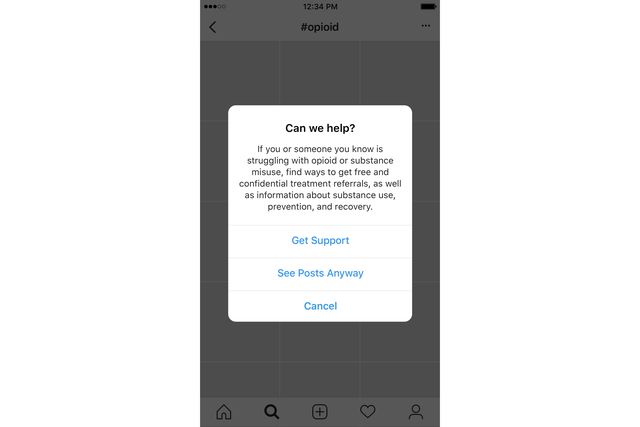The image depicts a dark gray interface of a website as viewed on a mobile device. At the top, it displays the time "12:34 PM." In the upper left corner, there is the hashtag "#opioid," while the upper right corner shows the battery life icon and three small dots symbolizing a menu.

In the middle part of the screen, there is a left-pointing arrow on the left side, and a pop-up box in the center with the message: "Can we help? If you or someone you know is struggling with opioid or substance misuse, find ways to get free and confidential treatment referrals as well as information about substance use prevention and recovery." Below this message, three options are presented in blue text: "Get Support," "See Posts Anyway," and "Cancel."

At the bottom of the web page, there are several icons representing different functions: a home icon for the main page, a search icon, a plus icon inside a square possibly for adding new content, a heart icon for likes, and in the lower right corner, a generic profile icon typically used for users who have not personalized their profile image.